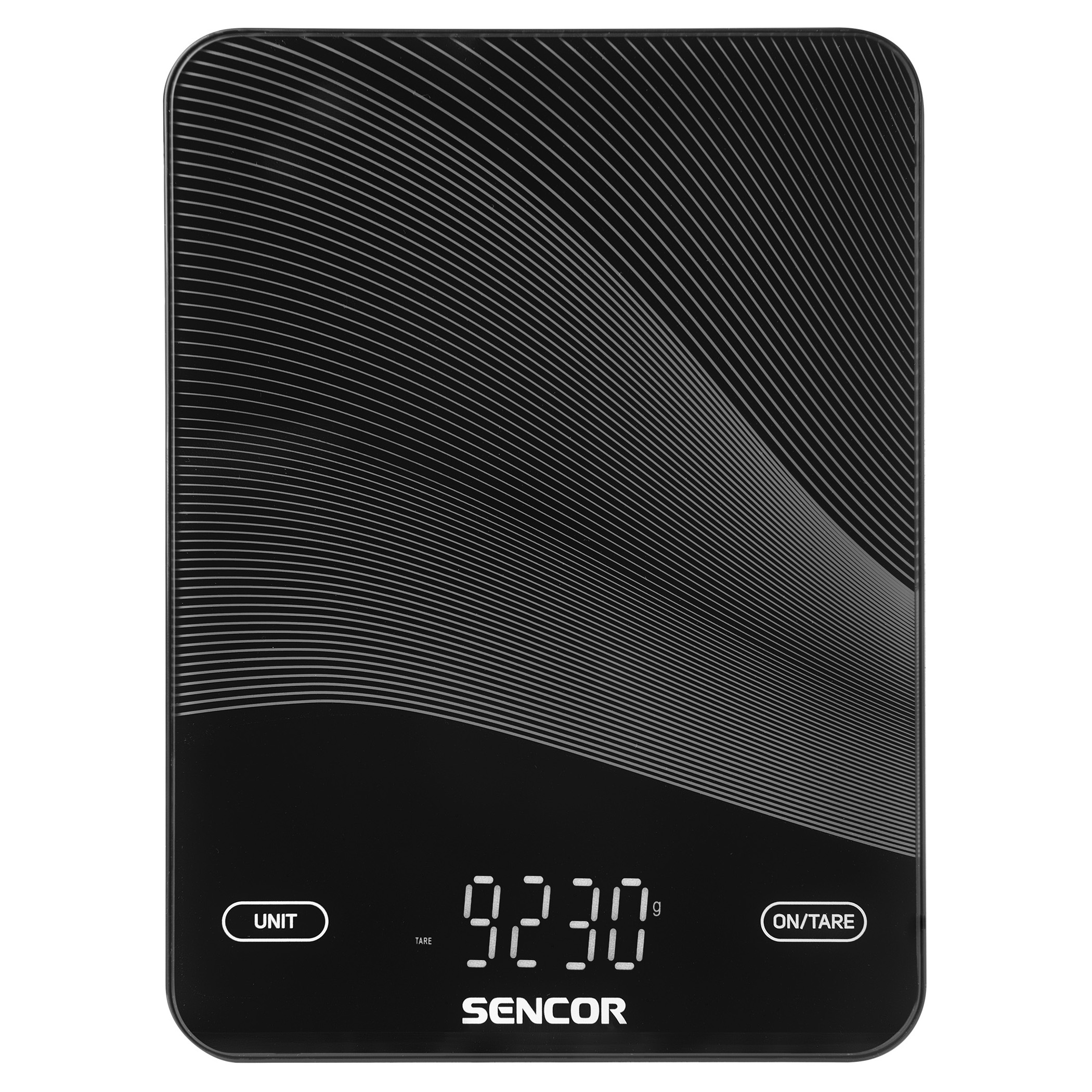This black and white image showcases the display screen of an electronic scale, likely from the brand SENCOR. The scale's rectangular design features rounded corners and a black background adorned with abstract decorations. At the top of the screen, there is an abstract design consisting of curved gray lines, with one band of tightly-packed lines appearing lighter, and a section of parallel lines on the upper right that are spaced further apart, giving a darker appearance.

The interface includes two oval-shaped text boxes at the bottom: the left one labeled "UNIT" and the right one "ON/T-ARE". Centrally displayed in the screen is the weight measurement "9230 g", with "g" indicating grams. The word "SENCOR" is prominently displayed below the measurement in white text on the black background. The scale appears to feature touchscreen buttons, designed for user interaction to toggle units or power the device, likely turning on automatically when weight is applied.